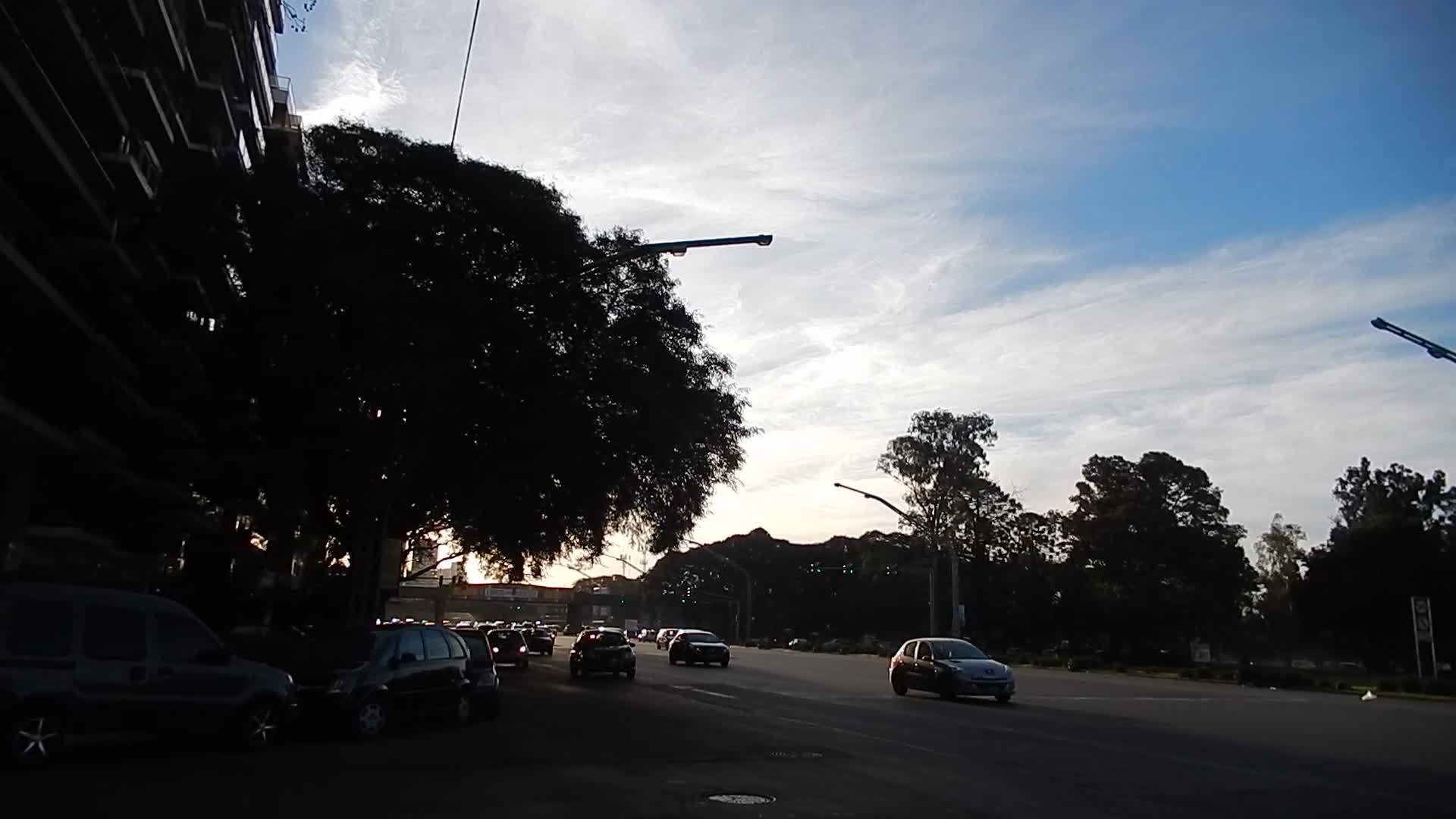This image captures a bustling urban scene taken from the side of a road in the late afternoon, just before nightfall. The sky is a deepening blue adorned with smooth, swirling white clouds. The photographer stands in the shadow of an apartment building on the left side, partly obscured by a large tree that also casts a silhouette. Directly in front of this tree, a few cars are parked, contributing to a small car park area. The road stretches ahead, busy with vehicles driving towards the camera. On the opposite side of the road, a row of trees stands silhouetted against the darkening sky, interspersed with light posts and telephone wires, enhancing the urban atmosphere.